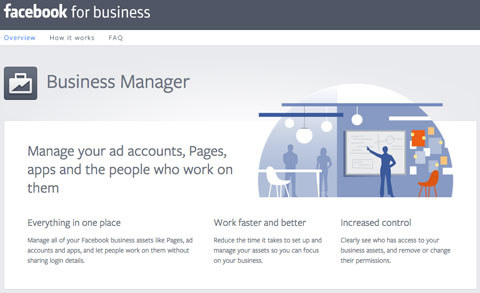The image features a predominantly monochromatic design with subtle color accents. It presents an overview of Facebook for Business, detailing how the platform works and providing a FAQ section. Prominently highlighted is the "Business Manager" tool, which promises streamlined management of ad accounts, pages, and apps, all centralized in one place to enhance efficiency and control. 

A graphical element includes an orange chair, two silhouetted figures interacting with a bulletin board, another silhouette seated next to a table, and additional essential office elements. The layout is divided into three main areas emphasizing the benefits of "Everything in One Place," "Work Faster," and "Increase Control." Interactive options invite users to explore further details on how the service functions and to access the FAQ section for additional questions.